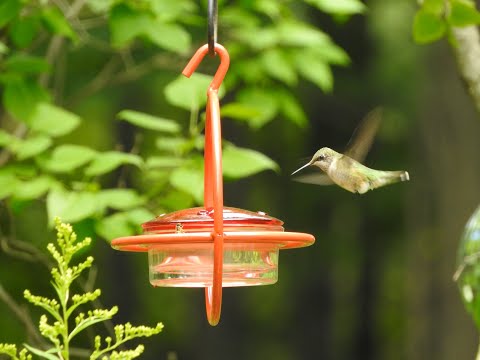In this image, a vibrant green and yellow hummingbird with a long beak is captured in mid-flight, its wings a blur, as it hovers just inches away from a red hummingbird feeder. The feeder, designed in a translucent short cylindrical shape with a red dome cap featuring multiple feeding holes, hangs from a black metallic hook. The setup includes a supportive framework reminiscent of thin metal, similar to that used in NFL face masks, encircling the feeder to keep it secure. The feeder is hanging in what appears to be a wooded area, with green leafy trees and plants visible in the background. Notably, on the bottom left corner, there is a plant with green leaves adding to the natural setting. This detailed setup creates an inviting scene for the hummingbird, ready to perch and sip nectar.